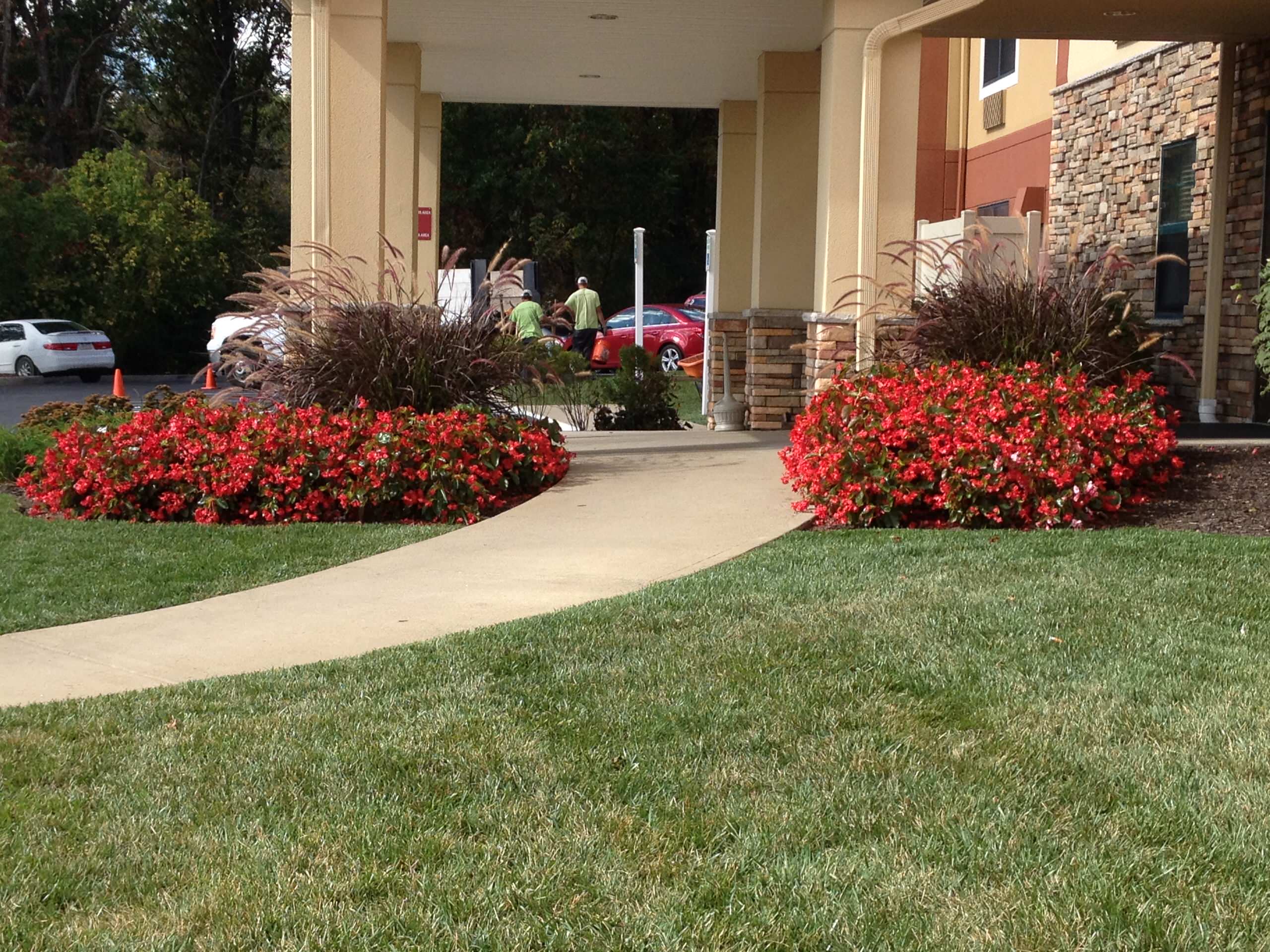The image showcases a meticulously landscaped area outside a modern building that might be a retirement home or hotel. The scene is centered around a beautifully manicured lawn and an off-white, curved walkway bordered with vibrant red flowers. Surrounding these flowers are bushels of tall, brown reeds creating a natural, garden-like atmosphere. In the background, you can see large trees adding a touch of greenery to the setting. The building itself features cream-colored pillars interspersed with intricate brickwork of various browns, slate gray, and white, creating a contemporary aesthetic. The walls also have red elements, adding to the modern look. Adjacent to this garden area, there's a parking lot containing two white cars and one red car, marked by two orange cones. Two people, dressed in green shirts and white hats, are walking away, possibly carrying bags. This scene captures a tranquil outdoor space blending nature with modern architectural design.